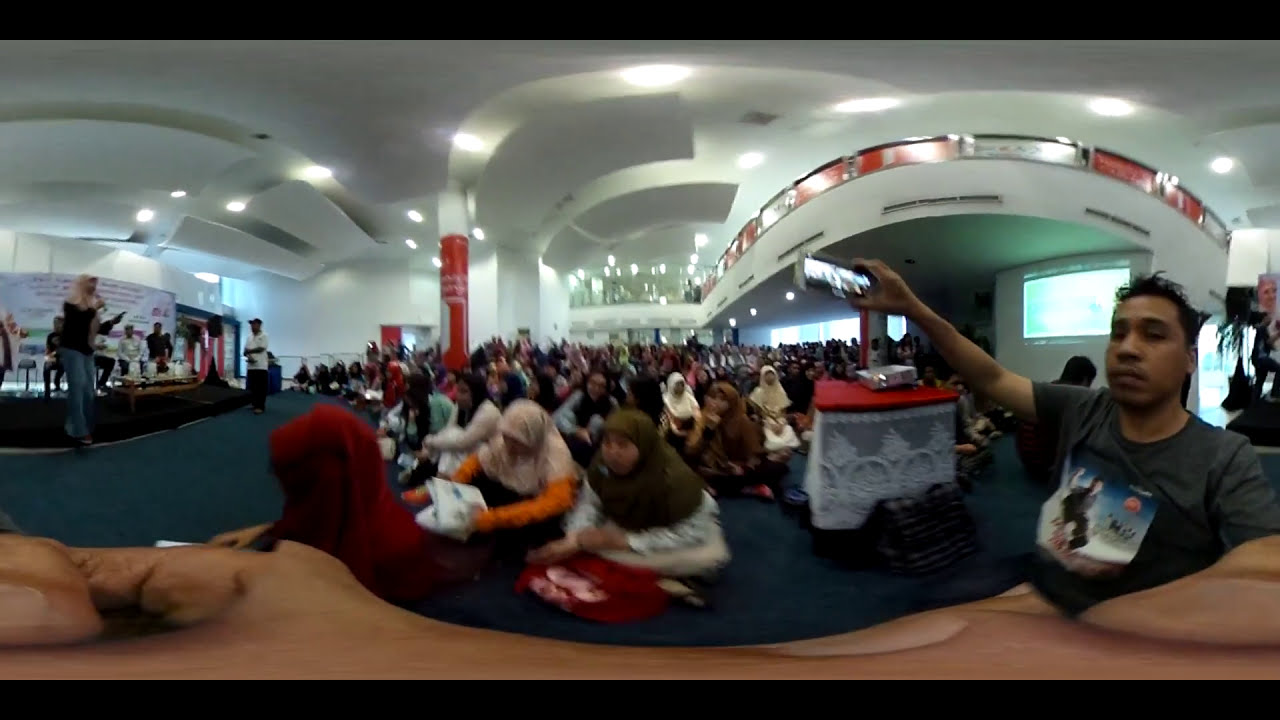The photograph, taken indoors, depicts a large conference or gathering, possibly exceeding 200 attendees, dominated by women wearing hijabs. The scene features a white arched ceiling, blue carpeted flooring, and a stage set with people. At the center, a woman wearing a hijab, a black sweater, and a blue skirt is holding a microphone and addressing the audience. Many women in the audience, also in hijabs, are seated on the floor, mostly facing the speaker, with rows extending back into the distance. To the right, a man with brown skin, short black hair, and a gray short-sleeve shirt, is seen holding a cell phone, possibly recording the session. The image has notable visual distortions, suggesting it might have been captured with a VR camera or is a composite of multiple photos. This results in some surreal warping, especially noticeable around the man's arm and the ceiling, creating an unusual and somewhat disorienting visual effect.